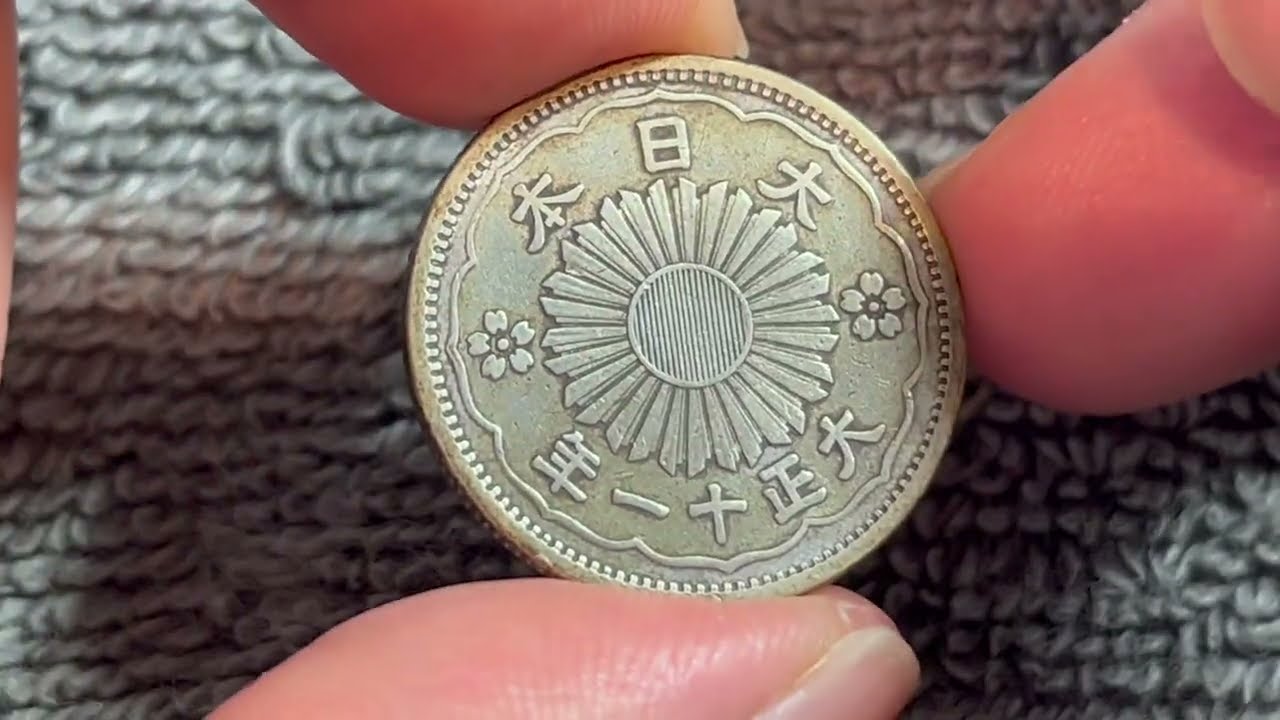In the image, a light-skinned person is delicately holding a coin between their two fingers and thumb, emphasizing the coin's intricate details. The coin itself, a faded goldish color with a hint of white, features a central circle with radiating bars, reminiscent of a sunflower. This central motif is surrounded by Asian characters, possibly Japanese or Chinese, with additional floral designs flanking the sides. The rim of the coin is detailed with a pattern resembling a zipper's teeth. The background is blurred but appears to be a gray fabric, perhaps a fleece or Sherpa blanket, which contrasts with and draws attention to the coin and the fingers holding it.